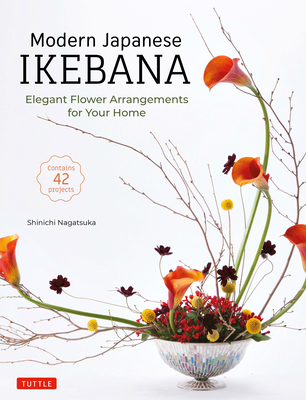The image depicts the cover of a book titled "Modern Japanese Ikebana: Elegant Flower Arrangements for Your Home" by Shinichi Nagatsuka. The background is white with the main title in large black font at the top left corner. Below the title, in green font, it emphasizes the subtitle "Elegant Flower Arrangements for Your Home," and in orange font, it states "Contains 42 Projects." The author's name, Shinichi Nagatsuka, is displayed beneath this. A focal point of the cover is a floral arrangement in a white bowl with a pedestal, featuring a variety of long-stemmed flowers, including blooming orange flowers and other multicolored flora such as red, yellow, and dark purple. There are also sprigs of red and green shrubbery, as well as twigs and stems, some reaching off to the sides and yet others yet to bloom. At the bottom left corner, a red rectangle with the white text "Tuttle" is prominently displayed, identifying the publisher. The overall impression is one of elegant and diverse floral arrangements, fitting the theme of Ikebana.